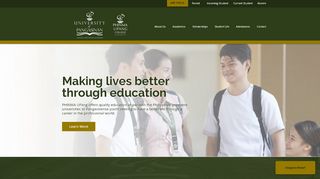A screenshot of a web page featuring a visually distinct layout and specific design elements. At the top of the page, the header displays "University of [Illegible]" in an olive green title bar. Within this bar are several white text links. Above the green title bar, the toolbar section includes a yellow rectangle with indecipherable text and four additional links aligned to its right.

The central portion of the web page showcases an image of school-aged teenagers. The students, dressed in white shirts and carrying backpacks with black straps, embody the educational theme of the page. Dominating the middle section is a prominent headline: "Making Lives Better Through Education." Below this, a descriptive paragraph outlines the mission or purpose of the website. Toward the bottom of the screenshot, a dark yellow button with the text "Learn More" invites users to engage further with the site's content.